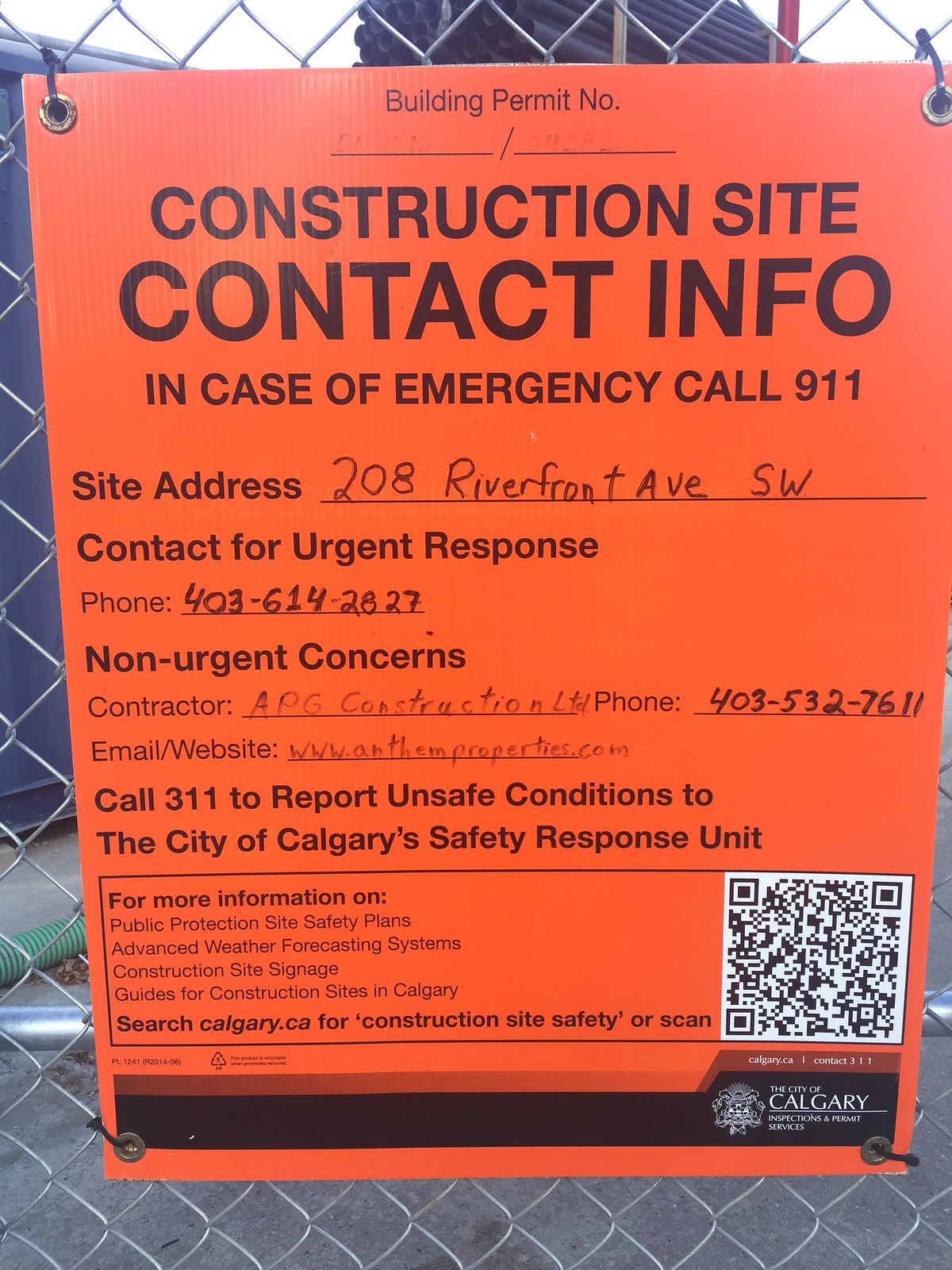This photograph shows a salmon-colored sign, zip-tied at the upper corners to a chain-link fence, with a construction site visible in the background. The sign displays important construction site information in bold, black, sans-serif uppercase font. The top of the sign reads "CONSTRUCTION SITE CONTACT INFO" followed by an emergency instruction: "IN CASE OF EMERGENCY CALL 9-1-1." Below this, there are several sections, some with handwritten details. The headings include "Building Permit Number" (the specific number is illegible), "Site Address" which is 208 Riverfront Avenue Southwest, and contact information sections. For urgent matters, it lists a phone number 403-614-2827, and for non-urgent concerns, it provides the contractor's details: APG Construction LTD, with a contact number 403-532-7611 and website www.anthemproperties.com. The sign also advises to call 311 to report unsafe conditions to the City of Calgary's Safety Response Unit. At the bottom, additional information about site safety and QR code for further details is displayed on the lower right side.